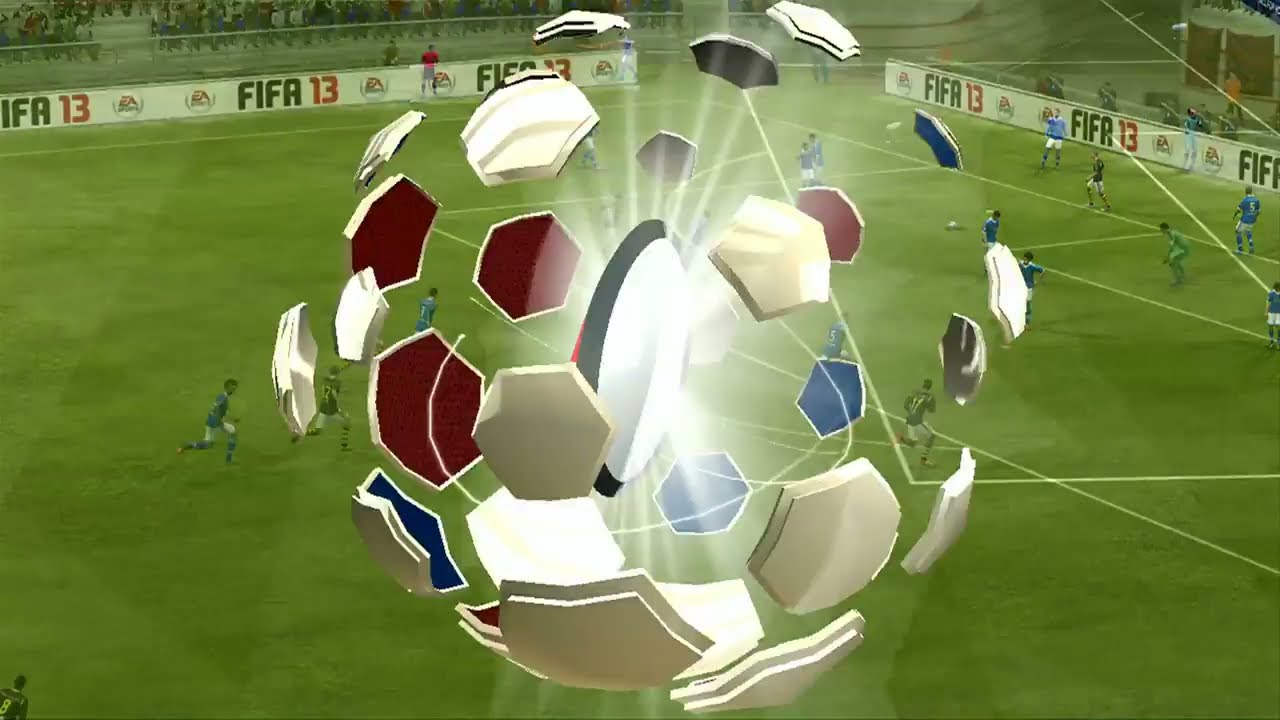The image captures a scene from a digitized soccer video game, featuring a vividly green soccer field. On the left side of the field, two teams are in mid-play: one in blue jerseys and white pants, and the other in black jerseys and white pants. The black team is pressing forward towards the goal, while the blue team defends. Notably, a blue player has fallen, and another blue-clad teammate rushes toward the ball from the right. Meanwhile, a black-shirted player, marked by a red arrow hovering above his head, is in close pursuit of the ball. The goalie, situated in the goal area on the left, stands poised and ready.

The scoreboard, located in the top left corner, displays "Air" leading with 3 points over "HOU" with 0 points, and a timestamp indicating 69:20 minutes into the game, implying the match has surpassed the standard hour. Additionally, prominent branding and text are visible: "EA Sports" at the top, along with a banner that reads "Go to easports.com," and another message, "GoalTrendSports.com," on the left. The game's HUD includes player names "Boateng" and "Diaf" at the bottom left and right corners, respectively. The central bottom part of the image features a mini-map of the field, detailing player positions. Also seen on the sidelines are several staff members, possibly including a referee and a cameraman, further enriching the dynamic scenario of this virtual soccer match.